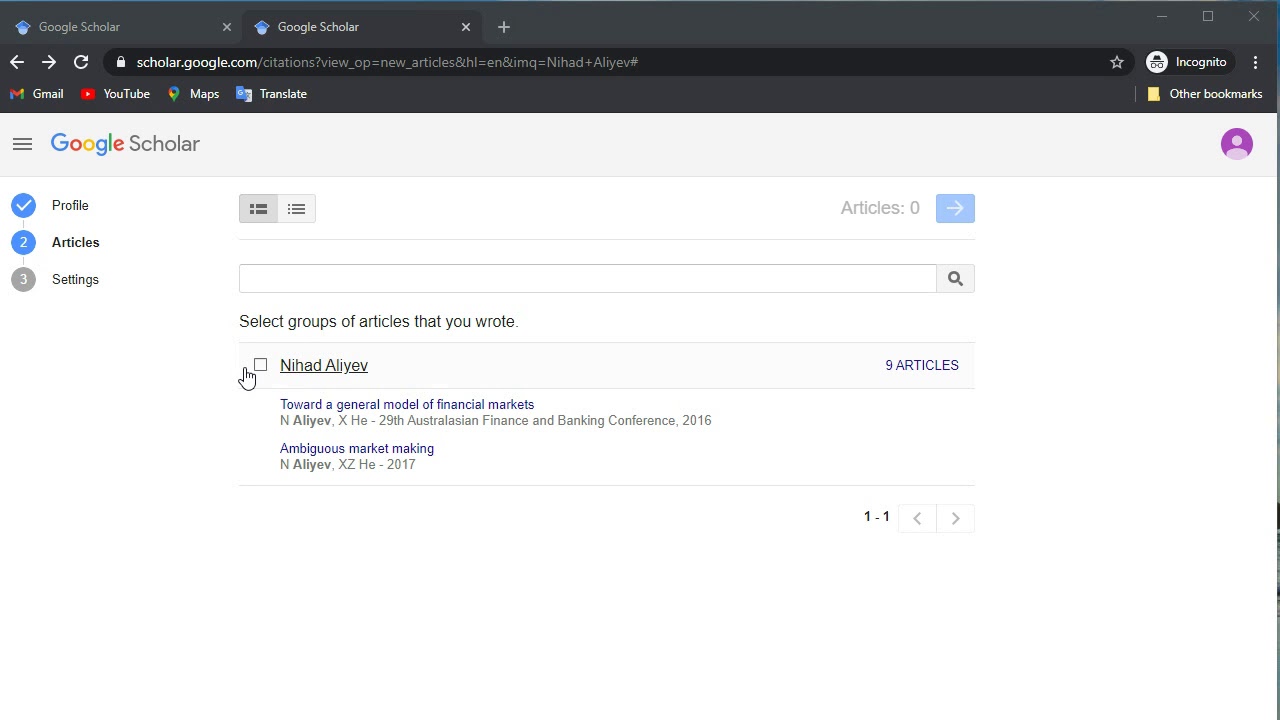The image displays a screenshot of a Google Scholar webpage. At the top left corner are two tabs labeled "Google Scholar." Below the tabs, the URL is visible against a black background, with the first 25% of the URL in white and the remainder in gray. Below the URL bar, a series of tabs are present, including Gmail, YouTube, Maps, and Translate. To the right, there is an icon indicating that the browser is in incognito mode.

The main body of the webpage has a light gray background. On the right side, there is a purple profile icon, while to the left, the "Google Scholar" logo is displayed, featuring the word "Google" in blue, yellow, and red lettering, and "Scholar" underneath it. The left-hand side of the webpage includes navigation links labeled "Profile," "Articles," and "Settings." 

To the right of these sections, there are gray and light gray squares, followed by the option "Articles" and a drop-down arrow. Below this, there is a section titled "Select groups of articles that you wrote," followed by the name "Nihad Aliyev." Underneath this, two links are visible with the search result status showing "1 of 1." The lower 75% of the image continues with a white background, providing a clean, minimalistic look to the interface.